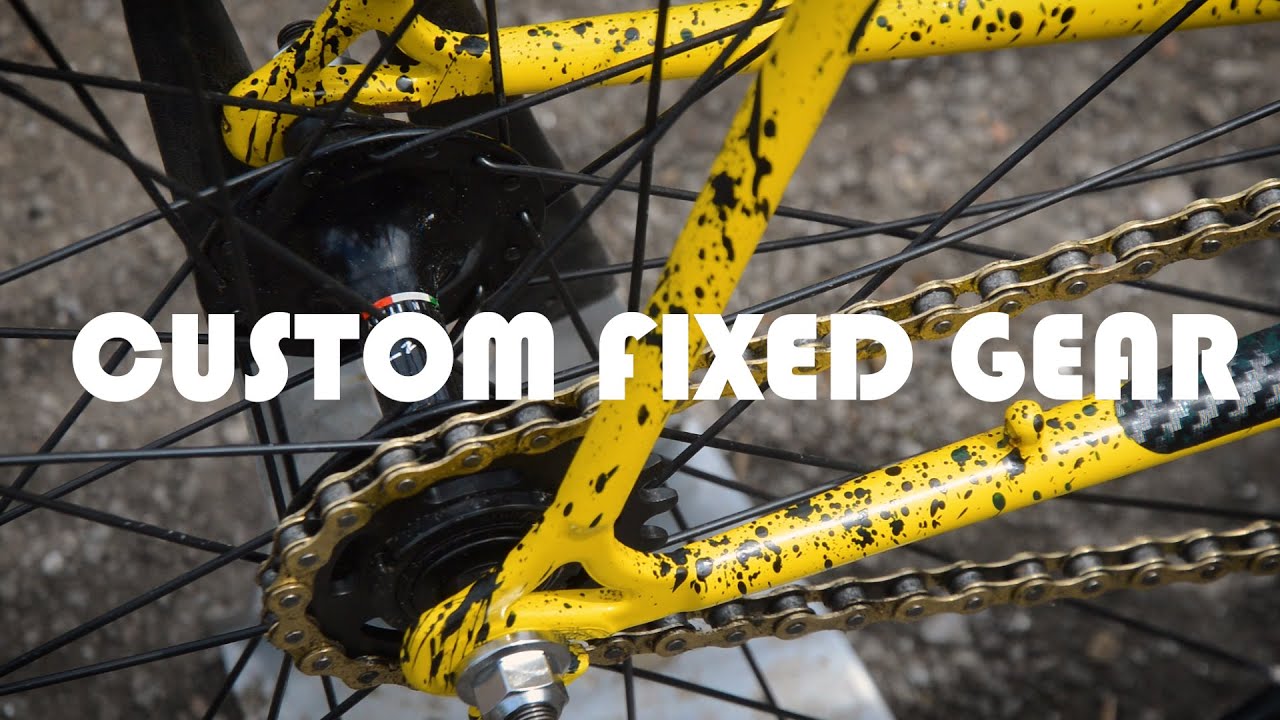The colorful advertisement features a close-up photograph of the rear wheel section of a custom fixed-gear bicycle. Dominating the image is bold white text in a rounded, chunky font stating "CUSTOM FIXED GEAR." The bicycle's frame is painted in a distinct school bus yellow with a black splatter pattern that evokes a Jackson Pollock style. This pattern could either be intentional or an accumulation of dirt, adding to the bike's unique aesthetic. Visible components include the black spokes and rims of the wheel, a meticulously clean gold chain looping around a small gear sprocket, and a carbon fiber section adorned with a subtle checkered black and gray design. A clean bolt and washer secure the axle, while the background reveals a ground surface that appears to be asphalt or gravel. There’s a tiny, hard-to-read red and white logo on the rear wheel, presumably the manufacturer's mark. This intricate snapshot encapsulates the gritty yet polished essence of a custom fixed-gear bicycle, seamlessly blending practicality with art.